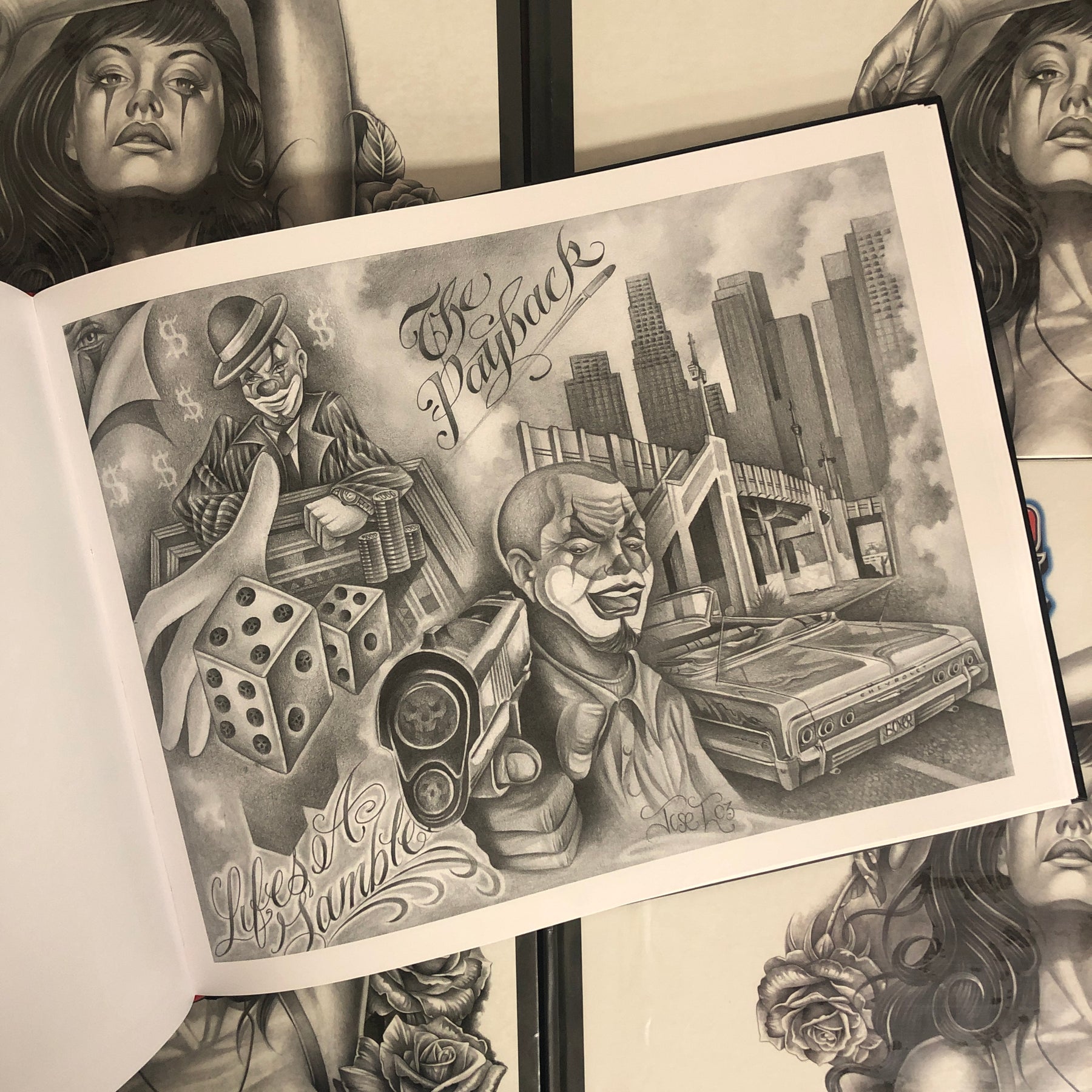The image depicts a stylized black-and-white illustration on a wide, rectangular book page, possibly a drawing book. Dominating the center of the page, a character resembling a clown is featured prominently in two scenarios: at the top left corner, he is engaged in a gambling scene with dice showing a roll of 5 and 4, and tokens scattered around, while dollar signs float above him. The man, adorned with clown makeup, is also seen at the bottom center of the image, pointing a gun directly at the viewer with a sinister smile, next to a car, against a backdrop of city skyscrapers.

Text elements on the page include "The Payback" in a stylized script at the upper center and "Life's a Gamble" at the bottom left. The background of the page is dominated by repeated black-and-white images of a woman with dramatic eye makeup and tears of mascara, her left hand positioned above her head, surrounded by roses. These details combine to create a complex, noir-esque composition that merges themes of risk, danger, and duality, evoking a sense of dramatic tension and storytelling.